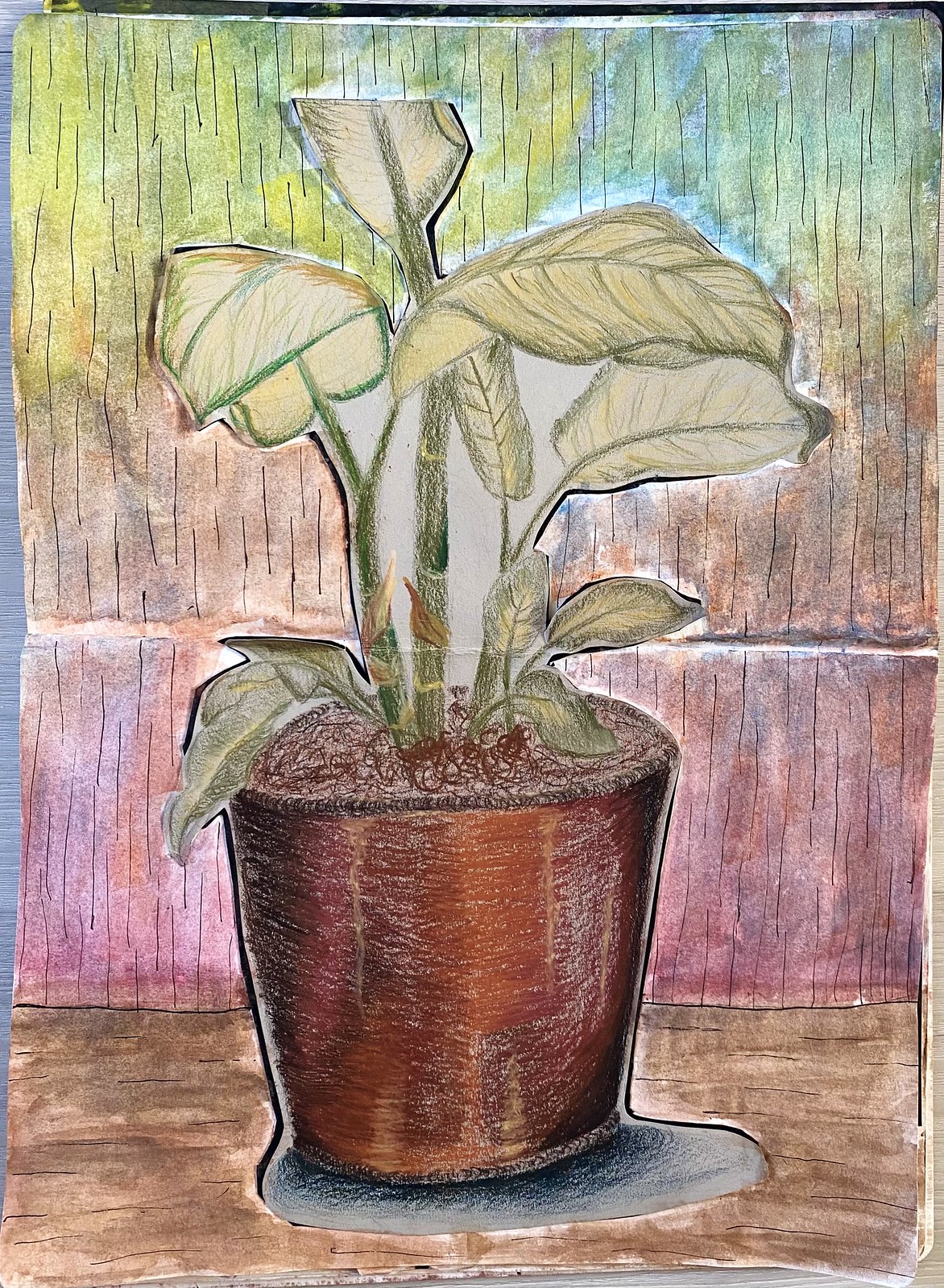The image captures a striking piece of art that blends different artistic styles and media, such as pastel colors and watercolor. The focal point of this artwork is an indoor plant with tall, pale green leaves featuring dark green veins, seated in a brown and maroon pot. The pot casts a distinct grey shadow on a wooden table below. The background is an intriguing gradient, transitioning from a maroonish hue near the bottom to shades of brown, yellow, green, and blue as the eye moves upward. The wall behind the plant is adorned with loose, top-to-bottom lines that merge the various colors in a harmonious, almost rainbow-like spectrum. The combination of detailed leaf shading and varied color transitions creates a unique, artsy composition that feels both playful and sophisticated, despite the artwork's somewhat naive execution, which suggests it may have been completed by a younger artist.